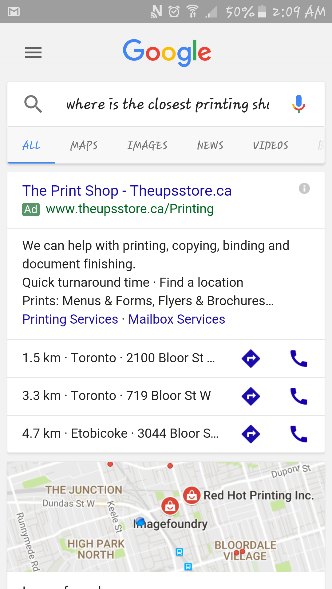The image is a screenshot of a Google search result on a smartphone, displaying the query "where is the closest printing shop." The page features a clean and functional design with a white background, typical of a Google search results page. At the top of the screen, there is a search bar with the query text.

Below the search bar, there's an advertisement for a printing shop from the website "theupsstore.ca/printing," highlighting services such as printing, copying, binding, document finishing, and quick turnaround times. The advertisement also mentions that they offer printing services for menus, forms, flyers, brochures, and mailbox services.

Underneath the advertisement, there are three location listings for printing shops, each including an address, distance from the user's location, and accompanying icons for phone calls and directions. The details are as follows:

1. **First Location:**  
   - **Distance:** 1.5 kilometers  
   - **Address:** 2100 Bloor St. W., Toronto, ON  

2. **Second Location:**  
   - **Distance:** 3.3 kilometers  
   - **Address:** 719 Bloor St. W., Toronto, ON  

3. **Third Location:**  
   - **Distance:** 4.7 kilometers  
   - **Address:** 3044 Bloor St. W., Etobicoke, ON  

At the bottom of the screen, there's a map displaying location markers for the listed printing shops, providing a visual representation of their proximity and exact locations. Each location marker on the map corresponds to the respective addresses listed above, allowing users to easily identify and navigate to the nearest printing shop.